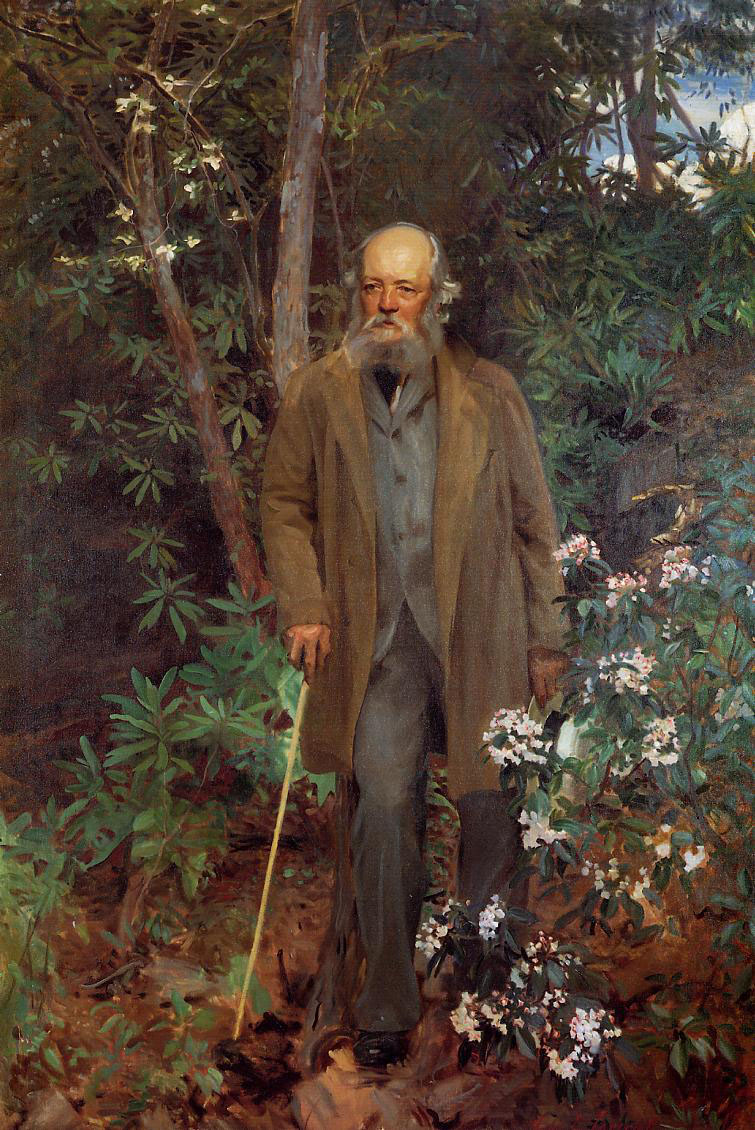In this highly detailed and photorealistic painting, an elderly man, probably in his 70s, is depicted walking through a dense wooded area. The man, centered in the middle of the image, faces towards the viewer, his intense facial expression and long white beard drawing attention. He wears a light brown jacket over a gray undershirt, gray pants, and black shoes, while holding a tan cane in his right hand for support. His balding head, with white hair on the sides, complements his distinguished appearance. Surrounding the man is an array of light green plants and white flowers, with brown dead leaves scattered on the ground. Above him, tree branches frame the scene, and a sliver of partly cloudy blue sky peeks through in the top right corner. The overall atmosphere suggests a serene, solitary walk through a lush forest, inviting curiosity about the man's backstory.